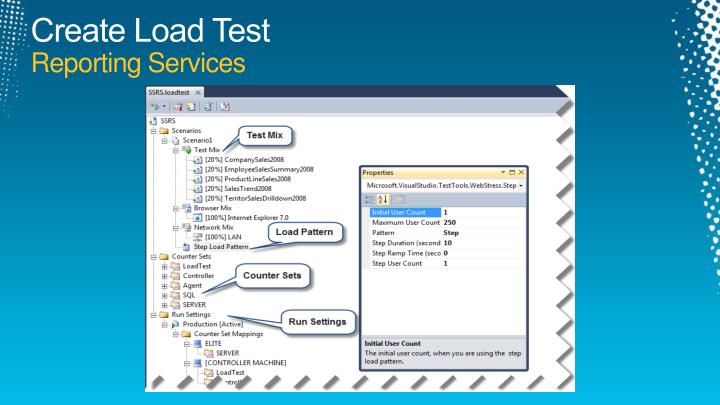The image is a screenshot of a computer application from a Windows machine, displayed in a horizontal rectangle. The background features a gradient effect, transitioning from light blue at the bottom to dark blue at the top, with a teal hue and scattered white dots on the sides. The focal point is a Windows program centered within the image, resembling a PowerPoint presentation slide.

In the upper left corner, there is a title that reads "Create Load Test Reporting Services." Below this heading, the graphical interface showcases a depiction of a complex file structure, with various documents and files listed. Several folders are expanded to reveal subfolders and additional contents, each accompanied by small text bubbles and arrows indicating more details. Key labels visible in the text bubbles include "Test Mix," "Load Pattern," "Counter Sets," and "Run Settings." Additionally, a pop-up window within the main interface specifies properties related to "Microsoft Visual Studio Test Tool Web Stress Steps," further emphasizing the detailed breakdown of information present. The application interface uses a color palette of teal blue, white, gray, black, yellow, green, and gold.